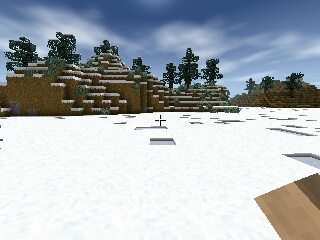The image depicts a whimsical scene from a cartoon-style video game. At the center of the screen is a prominent plus symbol. The background features rustic brown brick walls adorned with patches of snow, adding a touch of winter charm. Amongst the walls, small buildings contribute to the quaint, picturesque setting. Green-leaved trees with sturdy brown branches are scattered throughout, enhancing the village-like atmosphere. The ground, covered in white, square blocks, convincingly mimics a snowy landscape, tying in with the snow-topped bricks. Overhead, a clear blue sky dotted with fluffy white clouds completes the serene, enchanting environment.